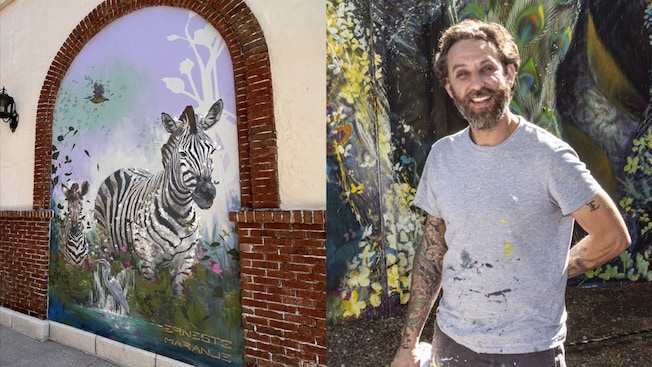The horizontally aligned rectangular image is divided into two distinct sections. On the left side, there is a mural inside a brick arch on a white concrete wall. The lower half of the wall is made of bricks, enhancing the architectural detail. The mural depicts two zebras, one adult and one young, standing in a vibrant green field filled with red and orange flowers. There is also a heron nearby and a background with a purple sky and large white flowers. The mural is signed "Erneste Moranje" in the bottom right corner.

On the right side of the image, a middle-aged man, presumably the artist, stands in front of another painted wall. He has light brown, curly hair mingled with gray, tan skin, and a beard. He is wearing a gray t-shirt splattered with paint and what seem to be brown pants, both stained with paint. He has intricate tattoos covering both arms; his left arm is tucked behind his back while his right arm hangs at his side. The ground beneath him is dirt with some yellow vines creeping up the wall behind him. The man's casual pose and smiling expression add a personal touch to the overall scene.